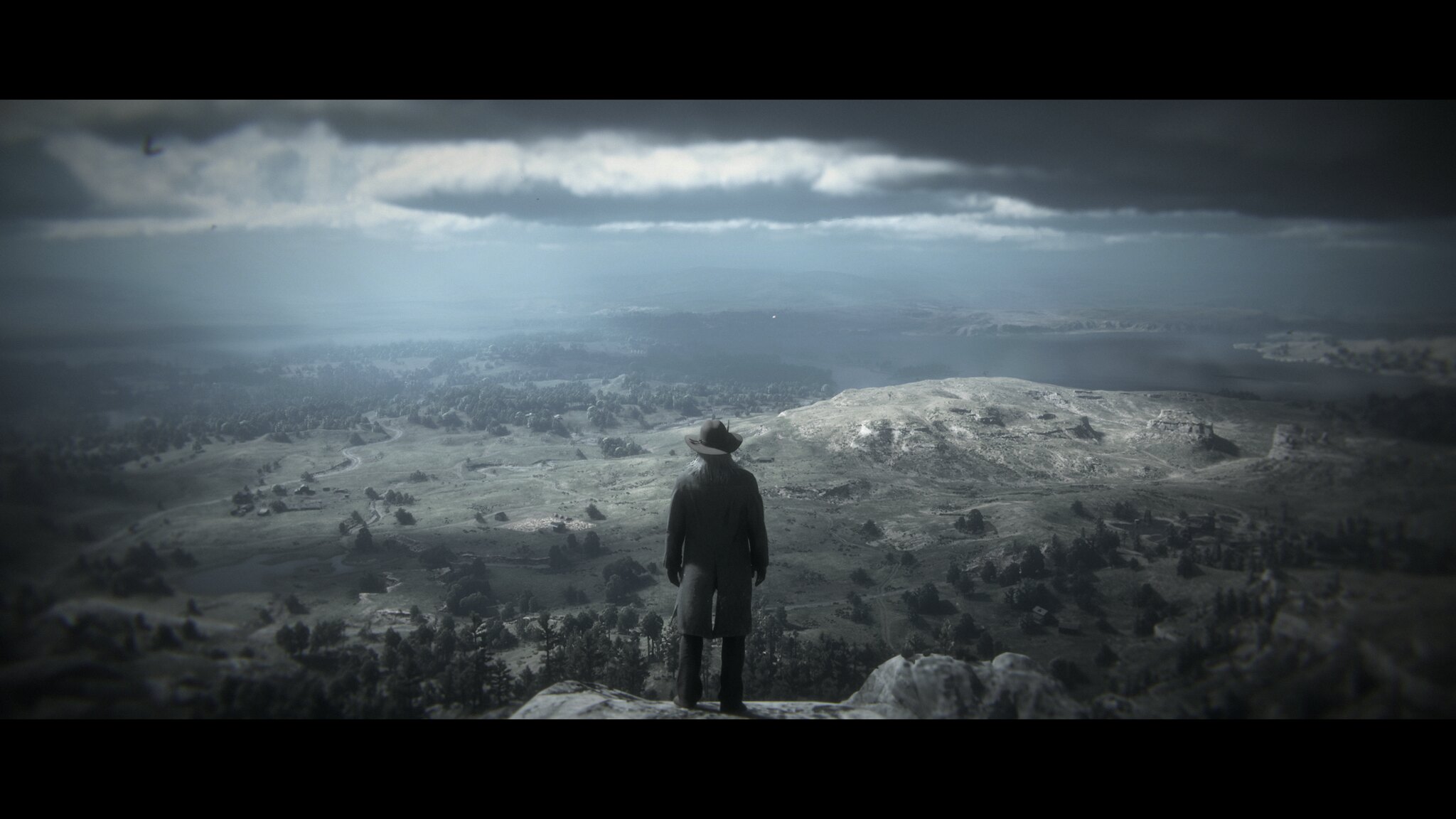In this screen capture from the video game Red Dead Redemption, a lone figure stands prominently in the center, embodying the quintessential Old West. The man dons a classic cowboy-style wide-brimmed hat and a long duster jacket, paired with pants that reach down to his sturdy boots. He is positioned on a rugged grey stone cliff that juts out over a sprawling, lush valley. The expansive landscape below is dotted with verdant green fields and an abundance of trees, interspersed with a few distant old buildings barely visible through the haze.

The atmosphere is shrouded in a somber mood, emphasized by the dark grey clouds overhead. Shafts of bright white light pierce through occasional breaks in the cloud cover, casting a stark contrast against the otherwise muted tones. The overall color palette of the image is dominated by greys and dark shades, contributing to a grim and desolate ambiance. This artistic choice enhances the dreary and foreboding essence of the scene, capturing the isolation and rugged beauty of the game's setting.